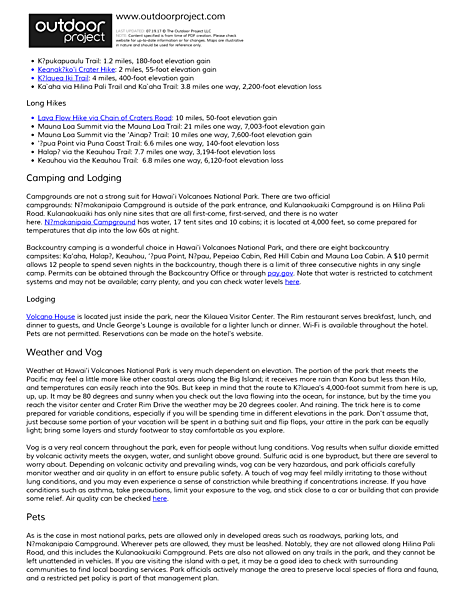This image is a screenshot from OutdoorProject.com. In the upper left-hand corner, there is a black box displaying the words "Outdoor Project." The rest of the webpage has a minimalistic design with a white background and black text, interspersed with blue hyperlinks.

At the very top of the page, the URL www.outdoorproject.com is visible. Directly beneath the URL, there is some text that is too small to read clearly. Below that is a section with headers and sub-sections where the actual content is formatted.

The first header reads "Long Hikes," and it is followed by six bullet points, each representing individual items or topics within this category. Next, the "Camping and Lodging" section appears, which contains two paragraphs of text. Within this section, there is a smaller subheader labeled "Lodging," accompanied by one additional, shorter paragraph.

Following that, another section is titled "Weather and Vlog," which includes two paragraphs. The final header on the page is "Pets," and this segment contains a single paragraph of information.

Scattered throughout the body of the text are eight blue hyperlinks, strategically spread across different sections, providing access to additional related content.